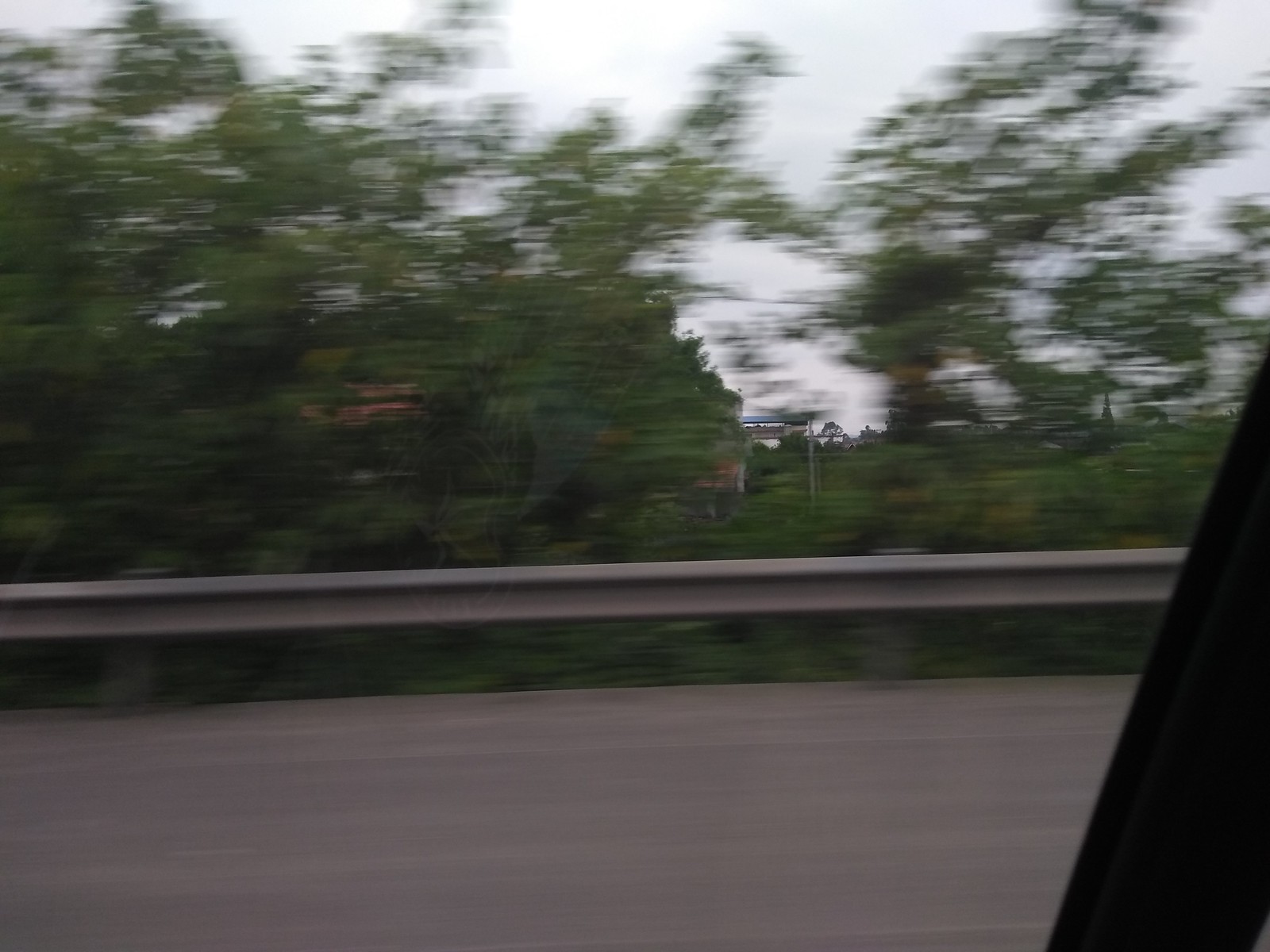Captured from the side window of a moving car, this photograph showcases a slightly blurred view of the road and the adjacent street, hinting at the motion of travel. The sky, painted in a soft light blue hue, bears an understated brightness as the sun subtly illuminates the scene, suggesting an overcast or early morning light. Off in the distance, a line of trees gracefully borders the horizon. Among them, you can discern the faint silhouette of a brick building, possibly a house or another structure, adding a touch of human presence to the landscape. Further beyond, a billboard looms faintly, barely perceptible against the backdrop, contributing to the sense of depth and the sprawling nature of the surroundings.